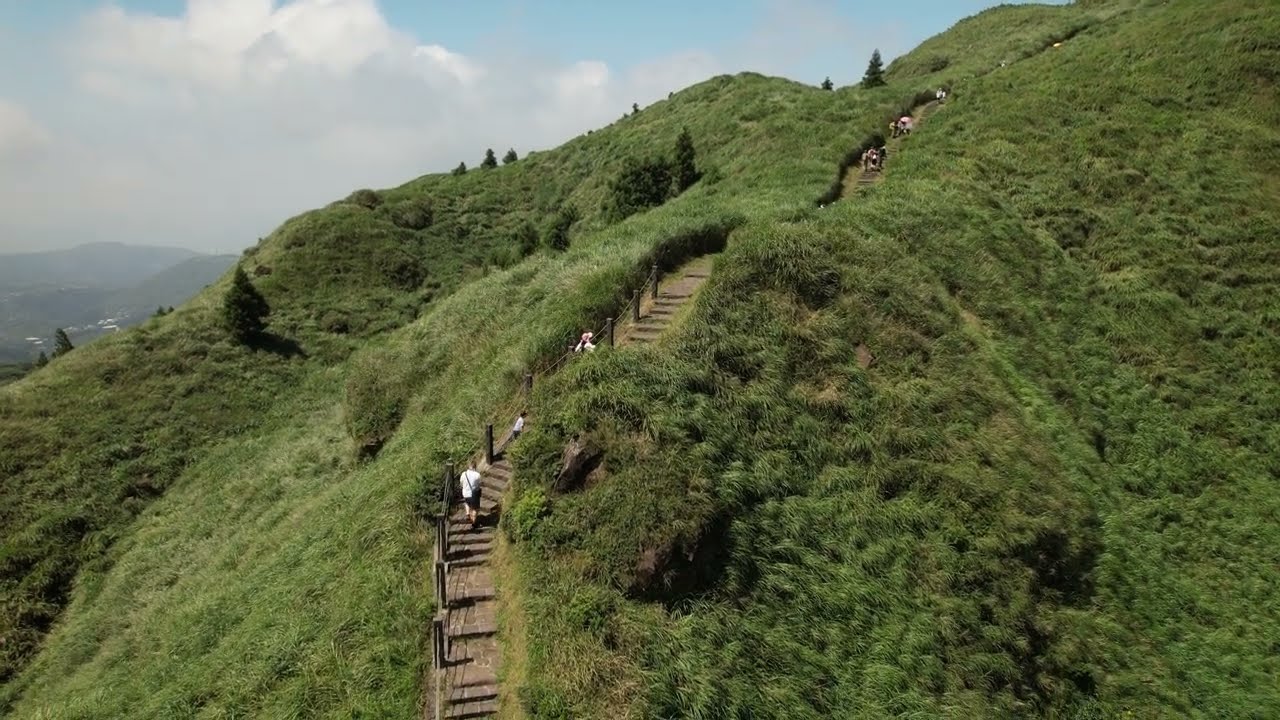This vivid drone shot captures a steep, winding pathway ascending a green mountainside covered in lush grass and dense vegetation. Amidst the greenery are nine short, bushy trees scattered across the hillside, adding to the picturesque scenery. The path, composed of wooden beams, chains, and brick steps, arcs up from the bottom center of the image to the upper right, reflecting the mountain's natural contour with its irregular curves and turns. Along the stairway, several people wearing white t-shirts and dark pants, some shouldering bags, can be seen making their way up the incline, while fewer are descending. In the distant background, larger trees and faint outlines of hills and buildings can be discerned, under a sky painted with light blue hues and dotted with fluffy white clouds and patches of grey fog. This serene yet dynamic landscape suggests that the path may lead to a vantage point like a temple or overlook, inviting hikers and nature enthusiasts to explore its beauty.